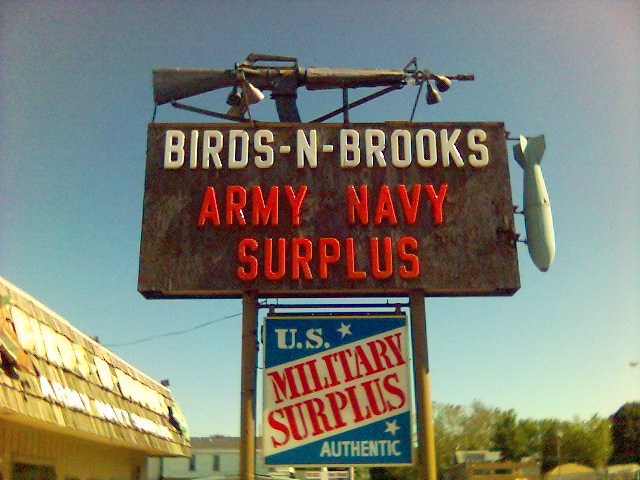A vibrant and detailed store sign catches the eye in this photograph. Mounted prominently atop the sign is a brown shotgun or hunting rifle with a sleek black handle, symbolizing the store's focus. Below this rustic firearm is a large, rectangular brown sign proudly displaying the store's name: "Birds and Brooks, Army Navy Surplus." Adding to the patriotic theme, a smaller tricolor sign in red, white, and blue declares, "U.S. Military Surplus Authentic". Enhancing the store's military-themed aesthetic, a small missile or rocket is attached to the larger sign, pointing downward. Framing the top right corner of the photo, a portion of a blonde wood roof peeks into view, further adding to the overall charming and nostalgic ambiance of the scene.